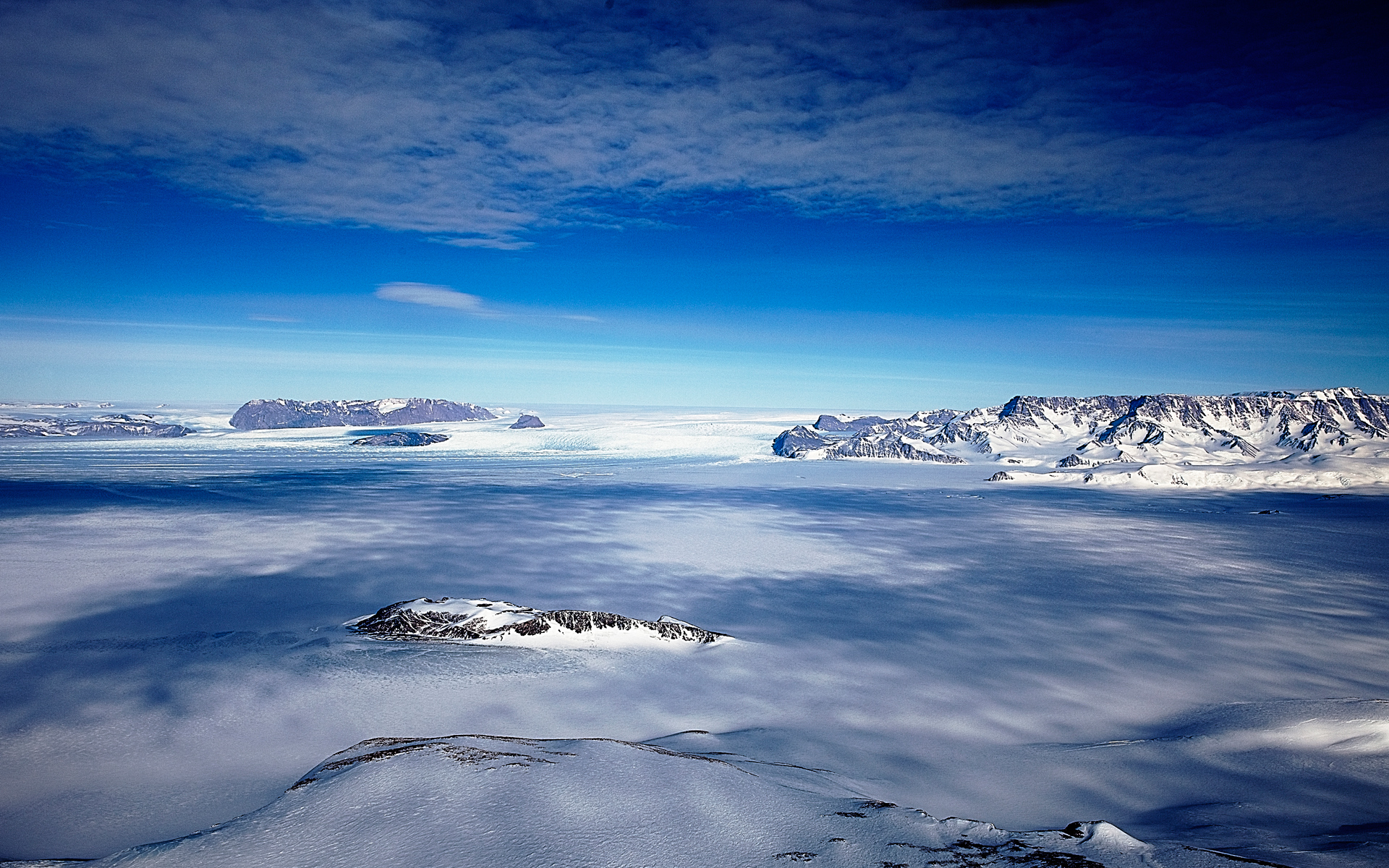This photograph captures a breathtaking panorama of a frozen wilderness, likely in the Arctic or Antarctica. Dominated by a rugged landscape where ice and snow interlace in a mesmerizing array of grays, blues, and whites, the scene portrays a dramatic, horizontal expanse of frozen earth or sea. Shadowed areas blend seamlessly with patches of lighter white, creating a natural tapestry of contrasting textures.

In the foreground, a smooth, snow-covered promontory serves as the vantage point from which the photograph is taken, cascading gently into the vast, flat snowscape that stretches towards the horizon. To the lower left, a small, gray, rocky mountain ridge punctuates the otherwise unbroken sweep of snow, nestled in a central valley-like stretch. Near the horizon, which bisects the image roughly halfway up the frame, a more prominent mountain range rises on the right side, while a smaller, fragmented range juts up on the left.

The sky transitions gracefully from a light blue at the horizon, intensifying into a vivid azure, and finally deepening into an almost inky black at the very top of the image. Sparse, flat gray clouds hang in the upper reaches of the sky, adding to the cold, isolated ambiance of the scene.